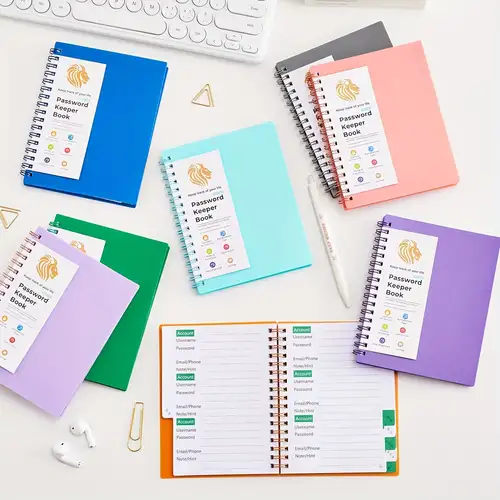A detailed photograph showcases an organized collection of multi-colored Password Keeper Books arranged on a desk. The desk setting features multiple accessories, including a white ballpoint pen, two AirPods, and both triangular and regular-shaped gold paperclips. The Password Keeper Books come in various hues such as blue, lavender, green, pink, gray, purple, aqua, and orange. Each notebook is spiral-bound and branded with a lion symbol and the text "Password Keeper Book," along with additional symbols indicating usage. 

The scene also includes a glimpse of a white keyboard in the upper part of the image, signifying a workspace environment. A notable detail is an open orange notebook, revealing lined sections and guidance for recording passwords. The books are meticulously positioned at different angles, with a deep blue notebook on the left side of the desk, piled atop a green and a light lilac one. To their right lies a light cyan blue notebook, and further to the right, a darker purple notebook adjacent to the open orange one. A peach notebook, stacked above a gray one, is visible on the right side of the image, completing the colorful array. This tidy arrangement, potentially part of a store display, emphasizes the functionality and organizational appeal of the Password Keeper Books.